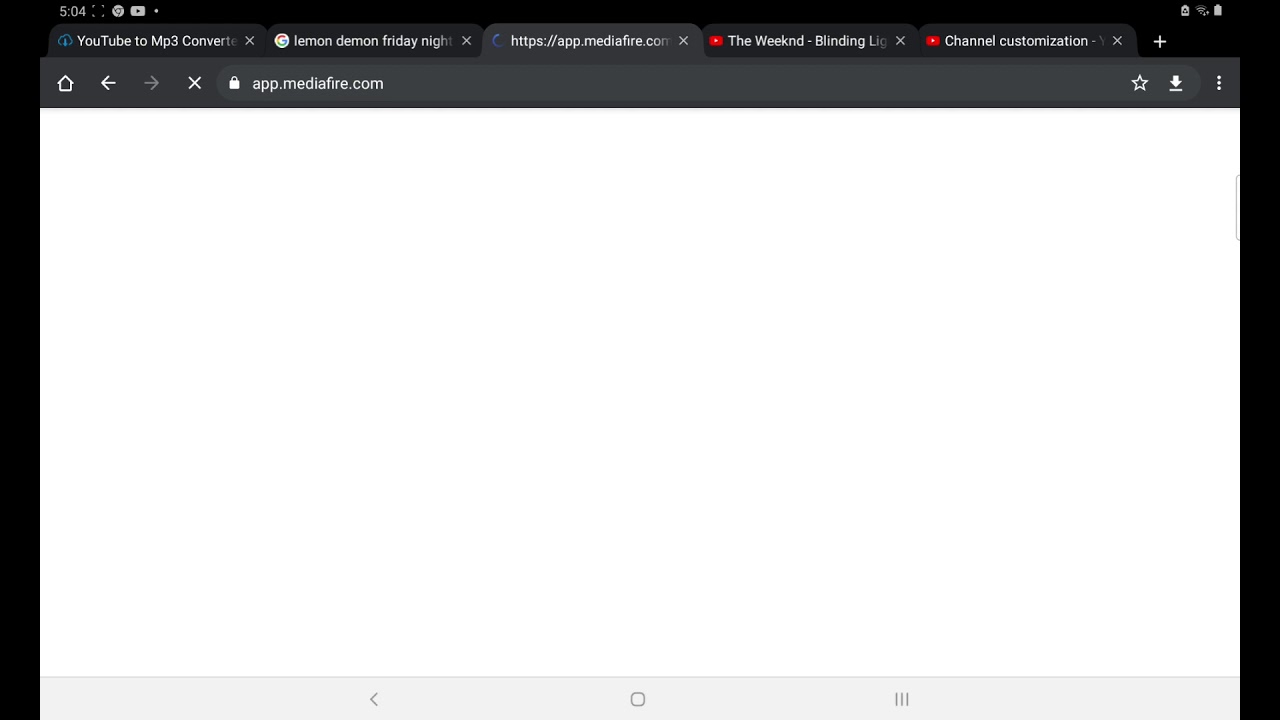This image is a cropped screenshot of a web page displayed on a tablet in landscape orientation. The tablet's background is black. At the top of the screen, there are five visible browser tabs, with the third tab selected. The URL in the search bar reads "app.mediafire.com." Below the address bar, the web page is entirely blank, presented as a white page, contrasting with the black browser interface.

At the bottom of the screenshot, a gray navigation bar stretches horizontally, featuring a left-pointing arrow for going back, a circular home icon, and a menu icon for minimizing screens. Additionally, the top right corner of the image displays device status icons, including the battery and Wi-Fi indicators.